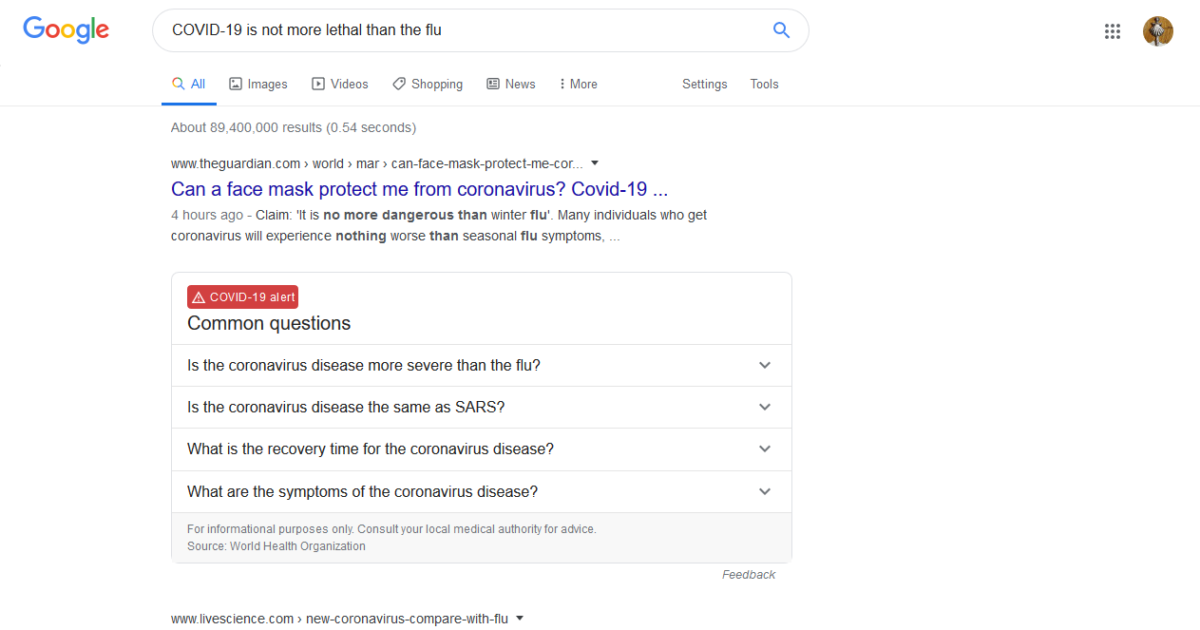This screenshot captures a Google search query conducted in the last few years, focused on the comparison between COVID-19 and the flu. The search term entered is "COVID-19 is not more lethal than the flu," with the search category set to "All." Adjacent categories such as "Images," "Videos," "Shopping," "News," "More," "Settings," and "Tools" appear grayed out, indicating they are not currently selected.

The search yields approximately 89,400,000 results in just 0.4 seconds. The first visible result, sourced from theguardian.com, poses the question, "Can a face mask protect me from coronavirus?" followed by a subtext stating, "COVID-19..." and "Four hours ago, claim." The claim discussed suggests that COVID-19 is no more dangerous than the winter flu, emphasizing that many affected individuals may only experience symptoms comparable to those of the seasonal flu.

Additionally, the page includes a "COVID-19 Alert" section containing commonly asked questions: "Is the coronavirus disease more severe than the flu?", "Is the coronavirus disease the same as SARS?", "What is the recovery time for the coronavirus disease?", and "What are the symptoms of the coronavirus disease?" These questions are dynamically generated by Google's algorithm to address popular user inquiries.

Towards the bottom of the screenshot, a partially visible result from livescience.com is noticeable. The interface appears to be formatted for desktop, featuring the classic Google logo prominently in the top left corner. The top right corner displays the user interface elements, including a notable amount of white space, a grid icon for Google apps (nine-dot menu), and a user profile picture. The profile image shows a man standing in front of a brownish wall.